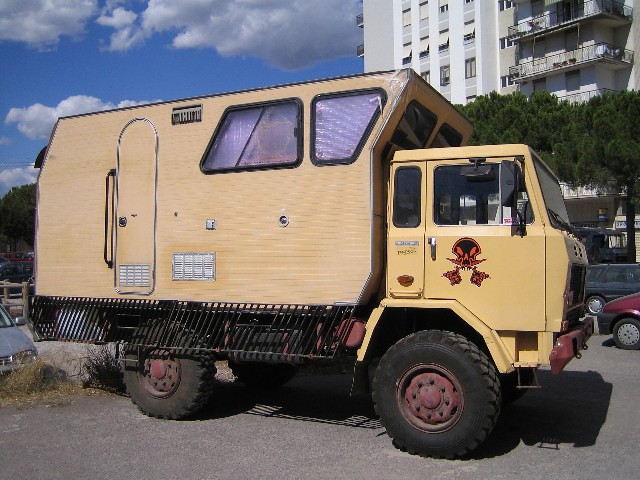This image features a distinctive yellow mini truck with an attached room or vanity van at the rear. The vanity van part features an oval (racetrack-shaped) door along with two illuminated windows that appear to have silver foil inside. There's also a small, narrow window at the top rear of the cab. Prominently displayed on the truck's door is a black decal of a scary, angry face with outstretched hands, accented in orange, and there's something hanging from the decal. The vehicle, which resembles a moving truck or RV, has large wheels that elevate the structure. The setup includes a rectangular door that might have stairs that pull out or a grating that lowers. There's a pair of vents visible on the side.

The truck is parked in a concrete lot adjacent to what looks like an apartment building with white walls. The surroundings include wooden fencing, trees, a parked car, and balconies with furniture. The bright blue sky dotted with white clouds adds a serene contrast to the otherwise functional scene.